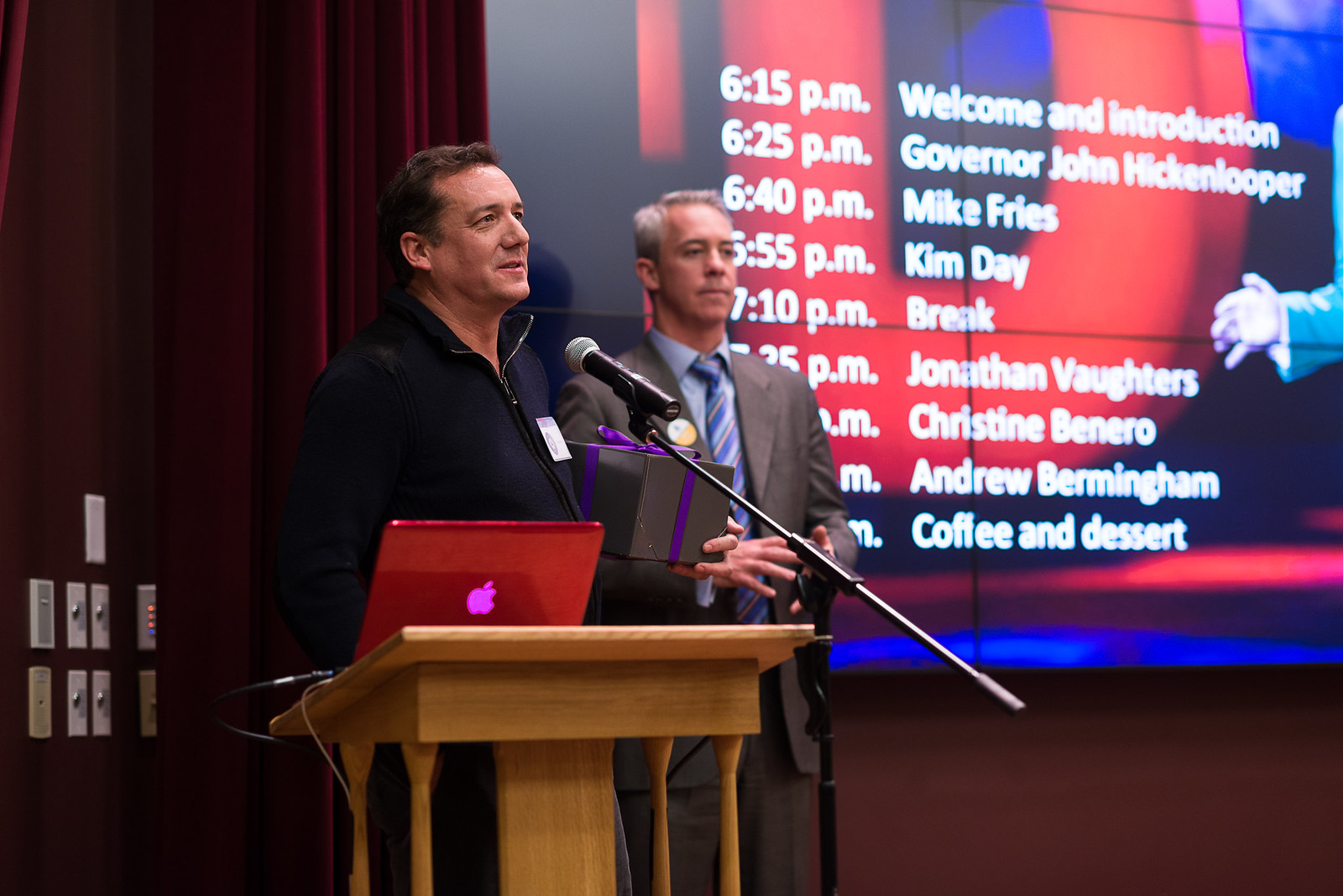In this image, two men are standing on a stage at a podium, appearing to give a speech. The man on the left, who looks middle-aged with brown hair, is speaking into a microphone. He has a red Apple Mac laptop situated on a wooden podium in front of him, possibly covered with a protective case. He also seems to be holding a gift wrapped with a purple ribbon. The man beside him, standing slightly behind, is dressed in a gray suit paired with a blue collared shirt and a blue-and-yellow striped tie, and has some gray hair.

Behind them, a screen displays an itinerary of the event, listing scheduled segments from 6:15 p.m. to the conclusion of the event. The itinerary details are:

- 6:15 p.m. - Welcome and Introduction
- 6:25 p.m. - Governor John Hickenlooper
- 6:40 p.m. - Mike Fries
- 6:55 p.m. - Kim Day
- 7:10 p.m. - Break
- 7:25 p.m. - Jonathan Voters (partially obscured)

Further items listed include Christine Berno, Andrew Birmingham, and the concluding Coffee and Dessert. The backdrop of the stage includes curtains and the projection screen.